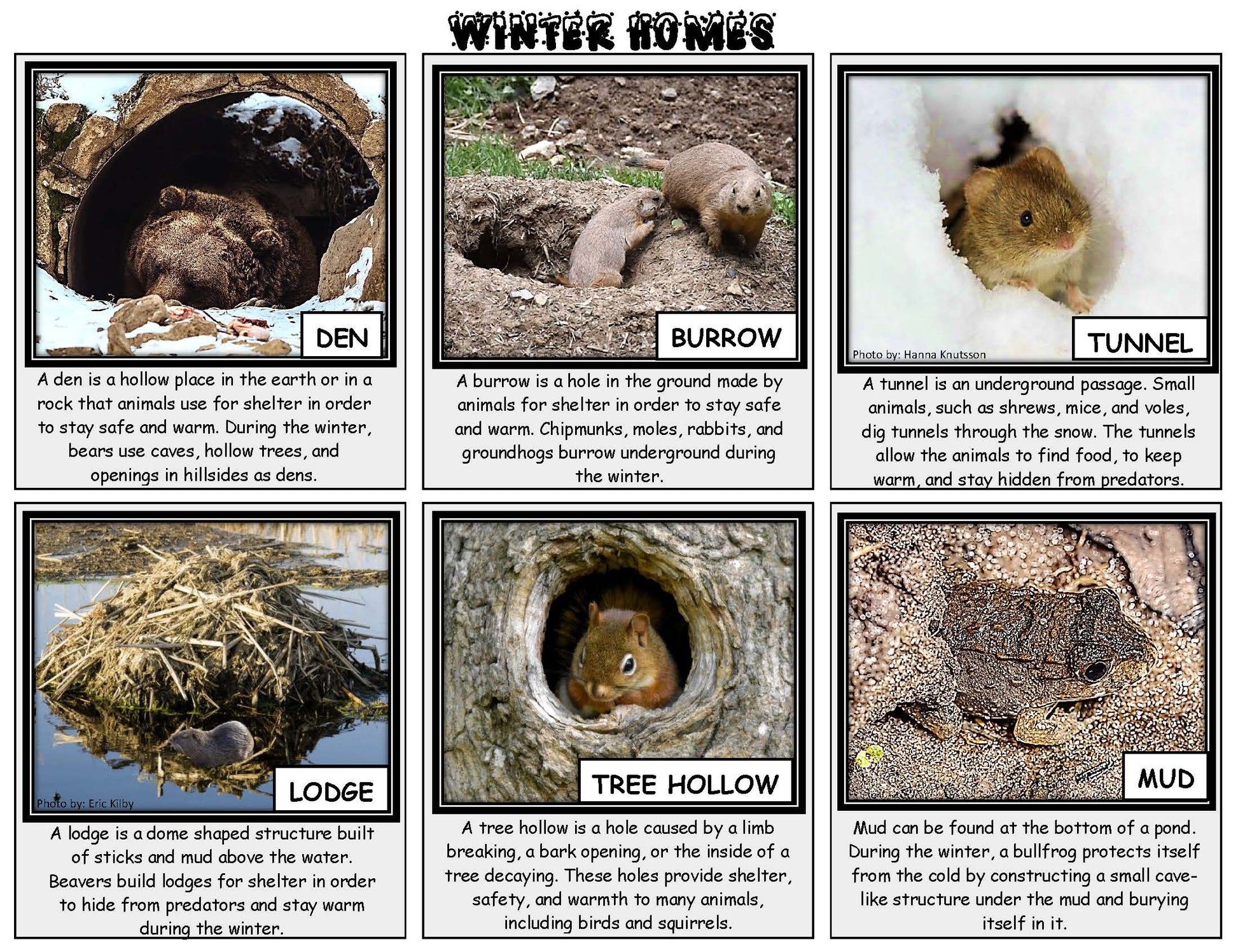The image, possibly from a book or magazine article about animal habitats, is titled "Winter Homes" in bold black text at the top against a white background. This landscape layout features six images arranged in two rows and three columns, each with a thick black border. The top row displays a snowy scene with a bear in a rock formation labeled "Den," animals climbing out of a ground hole labeled "Burrow," and a mouse peeking out of ice labeled "Tunnel." The bottom row features a pile of sticks in water with a beaver labeled "Lodge," a tree with a chipmunk in a hole labeled "Tree Hollow," and a frog in dirt labeled "Mud." Each of these vivid color photos includes a black-text description on a gray background, providing detailed explanations of these winter shelters, highlighting how different animals use them to stay safe and warm.